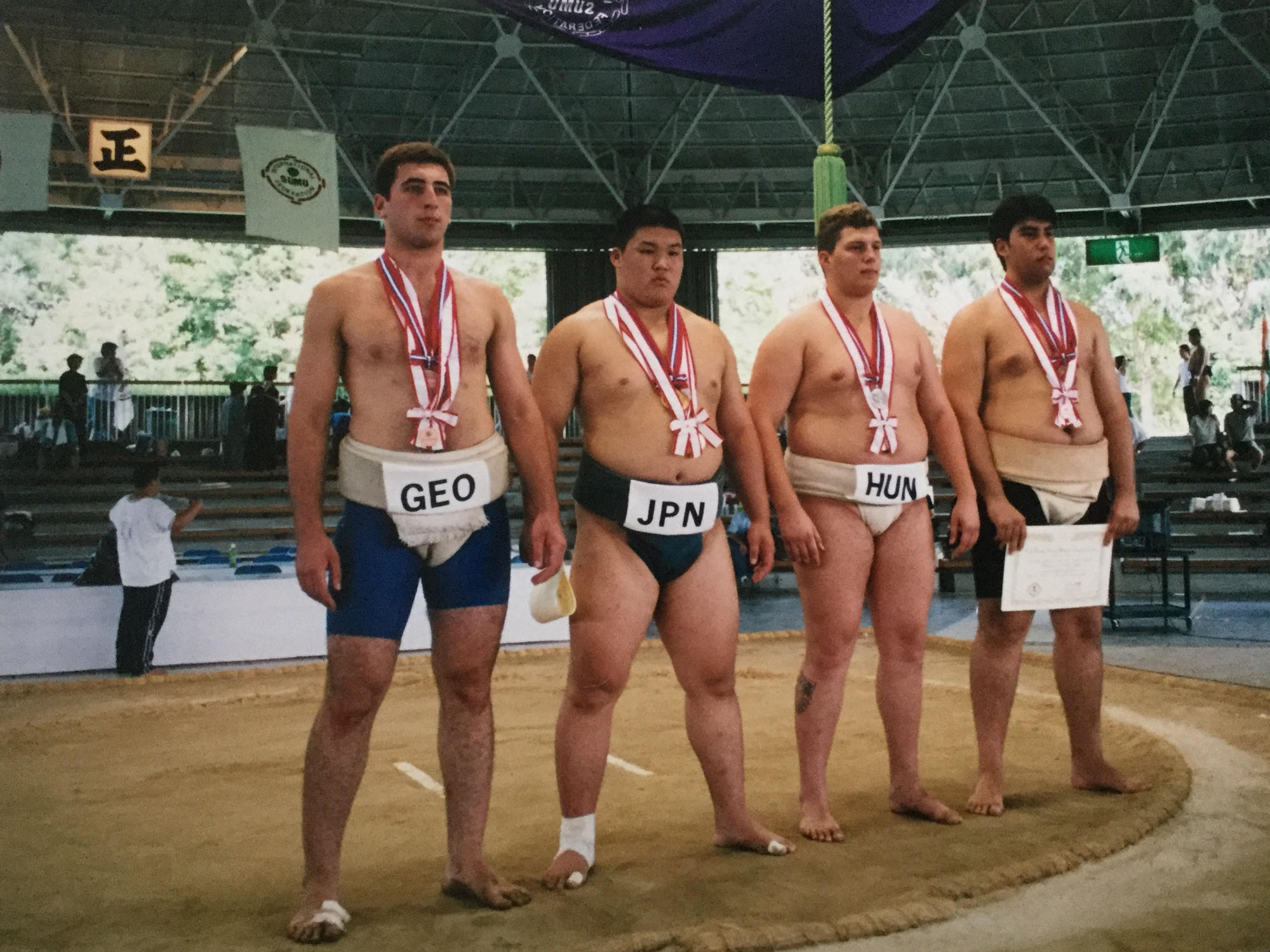In a small, semi-open arena set against a backdrop of lush green trees, a medal ceremony is underway. The arena features gray stands that rise only five or six levels, accommodating spectators who watch intently. The focus is on three shirtless athletes standing in what appears to be a sumo wrestling pit, dressed in tight bottoms appropriate for the sport. Each athlete is adorned with medals or ribbons, with vibrant red and white bands hanging around their necks. One athlete holds a sign that reads "GEO," another has a sign marked "JPN"—indicating Japan, while a third displays a sign that says "HUN," representing Hungary. In addition, one competitor holds a white certificate, though their country of origin is not visible. The ceremony captures a moment of triumph and international camaraderie amidst a rustic and intimate setting.